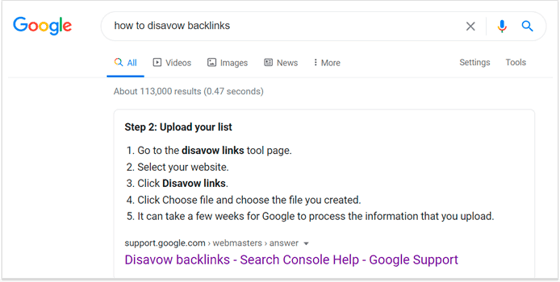The image displays a Google search results page with instructions on how to disavow backlinks. At the top left corner is the Google logo, featuring the following colors: a blue "G," a red "o," a yellow "o," a blue "g," a green "l," and a red "e." Below the logo are navigation tabs for "All," "Videos," "Images," "News," as well as additional options under "More," "Settings," and "Tools" towards the right.

The search results indicate approximately 113,000 results generated in 0.47 seconds. The top result provides a detailed, step-by-step guide to disavowing backlinks:

1. Go to the Disavow Links Tool page.
2. Select your website.
3. Click on "Disavow Links."
4. Choose the file you created by clicking "Choose File."
5. Note that it may take a few weeks for Google to process the uploaded information.

Below this guide, the URL path is displayed as "support.google.com -> webmasters -> answer," followed by a clickable tab. Additionally, there is a highlighted link in purple that reads "Disavow Backlinks - Search Console Help - Google Support."